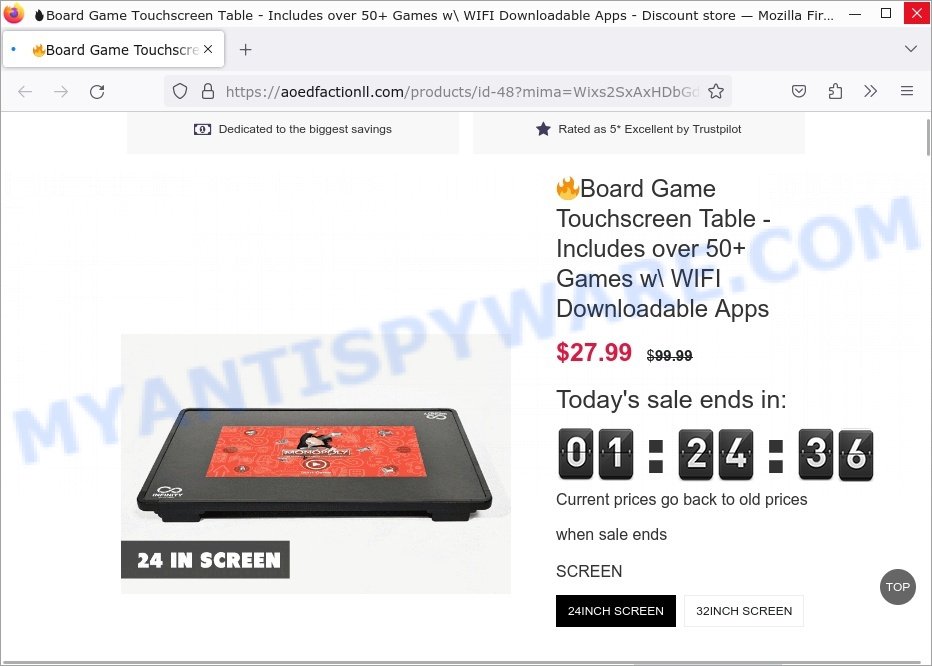The website has a white top border and features the Firefox symbol in the upper left-hand corner. Opposite this, there is a black flame icon, followed by the text "Board Game Touchscreen Table - Includes Over 50+ Games with Wi-Fi Downloadable Apps - Discount Store - Mozilla and Firmware…" in black. Below this, there is a white tab labeled "Board Game Touch..." and further down, the website URL "aoedtactionll.com" is displayed.

Adjacent to this are two gray rectangles side-by-side. The left rectangle reads "Dedicated to the Biggest Savings" in black text, while the right one showcases a "5-star Excellent" rating by Trustpilot.

On the right side, the text repeats "Board Game Touchscreen Table - Includes Over 50+ Games with Wi-Fi Downloadable Apps," and highlights in red the price "$27.99" (previously "$99"). The offer includes a countdown timer in white text with a black border: "Today's sale ends in 01:24:36." The product features a 24-inch screen, with a note that prices will return to the original amount when the sale ends.